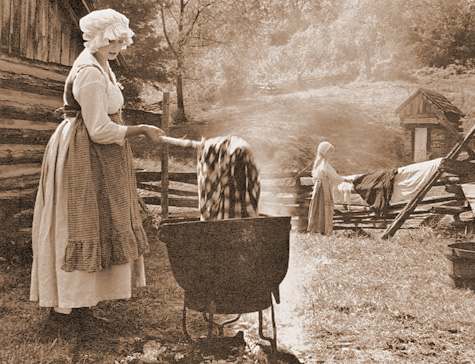The image is a detailed black and white photograph, possibly taken in the 1800s or early 1900s, with sepia overtones, depicting two women engaged in laundry work on a farm. The woman in the foreground is dressed in period attire, including a white bonnet, a checkered apron, and a long white dress. She stands beside a large iron cauldron where she is using a stick to stir and lift pieces of fabric, possibly shirts or linen, from the heated water. Behind her, another woman is seen hanging laundry to dry over a wooden fence. The scene is set outdoors with a barn to the left, trees and hills in the background, and a small log cabin or outhouse structure visible to the far right. Both women are immersed in the tasks of washing and airing out the clothes, indicating a moment of daily farm life during that era.